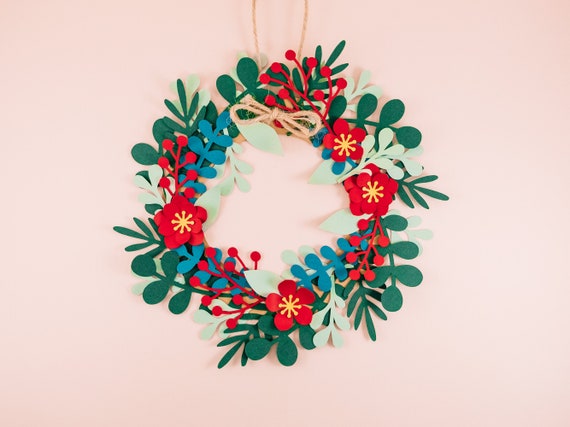The image features a festive wreath against a pale pink background. This intricately crafted wreath is not made from real natural materials but instead composed of various cutouts from felt or construction paper. The wreath is adorned with vibrant red flowers that have yellow centers, contributing to its lively appearance. Surrounding the flowers are an array of leaves in different colors: deep blue, light olive, dark green, and pale mint green. Additionally, red and teal-green leaves add to the rich diversity of the piece. The top of the wreath is accented with a natural-looking rope bow, from which two pieces of twine extend, potentially for hanging. The carefully arranged design includes a pattern where each flower is accompanied by red, blue, olive, and dark green leaves, creating a harmonious and festive decoration.